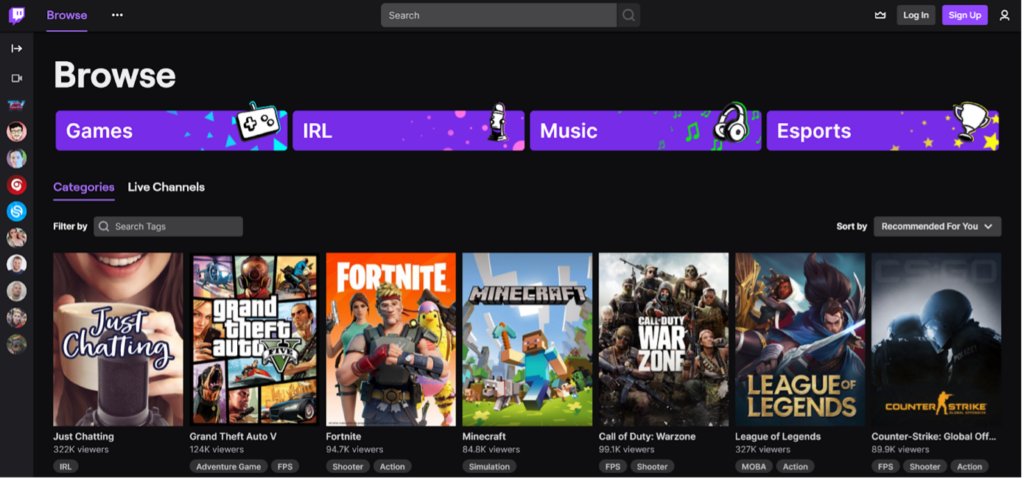The image depicts a detailed landing page for Twitch. At the top, the Twitter logo is represented within a purple box designed like a chat bubble, featuring a white box overlay and two purple lines emblematic of eyes. On the right side of the header, the word "browse" is highlighted in purple, indicating it’s selected, alongside a dark gray rectangle containing three white ellipses.

Central to the header is a dark gray search bar with light gray "search" text, adjacent to a black square housing a dark gray magnifying glass icon. Towards the right, a white crown icon is visible followed by two buttons: a dark black "login" button with white text, and a purple "sign up" button with white text. Further to the right is a human silhouette icon.

Within the navigation area, the word "browse" is prominently displayed in bold white, accompanied by multiple category buttons. The first button, in purple, labeled "games," features a white game controller icon flanked by cyan blue triangles. The subsequent button, labeled "IRL," showcases hot pink dots, followed by "music," incorporating a pair of white headphones and teal music notes. The final button in this row is "esports," characterized by a trophy icon set against a backdrop of yellow stars.

A series of various Twitch webpages are illustrated below, beginning with a woman smiling and holding a cup of coffee beside a microphone, categorized under "Just Chatting" with 322K viewers. This category is tagged as IRL. 

Next, "Grand Theft Auto V," an adventure and FPS game, shows 12.4K viewers. Following it, "Fortnite," labeled as a shooter and action game, has 94.7K viewers. Adjacent to it, "Minecraft" with 34,800 viewers is labeled as a simulation game. 

Proceeding to "Call of Duty: Warzone," this FPS and shooter game shows 99.1K viewers. Further down, "League of Legends," a MOBA and action game, has an impressive 327K viewers. Finally, "Counter-Strike: Global Offensive" is presented with 89.9K viewers, categorized as an FPS, shooter, and action game.